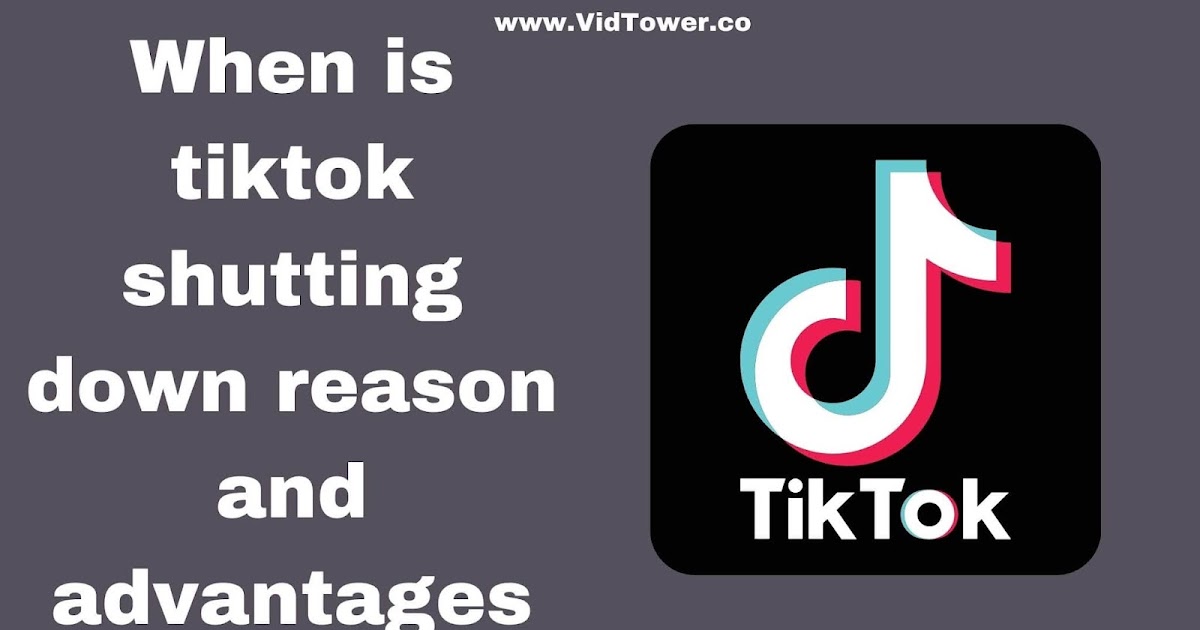A detailed screenshot captured from what appears to be a video, possibly a slide or a frame from a TikTok-related advertisement. The image is rectangular and set against a dark gray, almost off-color gray background. Centered at the very top is the text "www.vidtower.co." On the left side of the screenshot, there's a block of text that reads, "When is TikTok shutting down, reason and advantages." To the right of this text block is the TikTok app icon, which matches the familiar mobile device logo of TikTok. The icon is placed within a square with rounded corners and a black background. The TikTok logo, consisting of a stylized 'd' with a curve extending to the right at the top, is displayed prominently. The logo features multiple colors, including teal, white, and neon red, and the word "TikTok" is situated below it. Overall, the exact nature of the content is unclear, although it might be a part of a video, an ad, or a frame discussing TikTok's potential shutdown and related information.